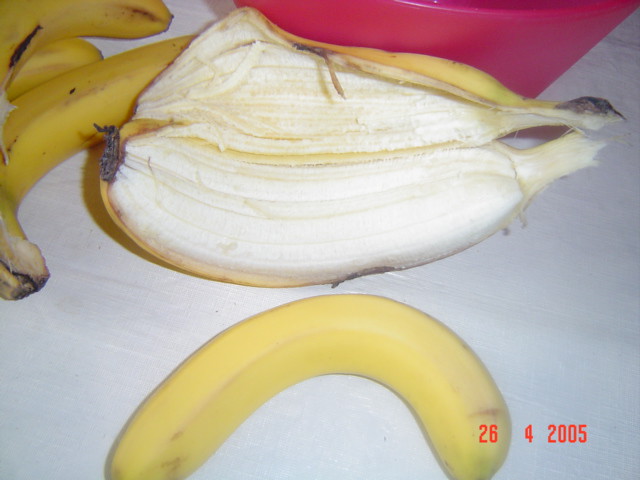This photograph, taken on April 26, 2005 (as indicated by the date stamp in the bottom right corner), showcases an assortment of bananas arranged on a white surface, possibly a tablecloth or plastic. In the composition, a peeled banana peel stretches horizontally in the middle of the frame with its sections spread open, reminiscent of an opened box. Below it, a banana rests on its side with its curve creating the semblance of a frown. In the upper left corner, three more bananas are partially visible, with the most prominent one lying closest to the peel. A red object, possibly a bucket, is positioned behind the opened peel, adding a splash of color to the predominantly yellow and white scene.